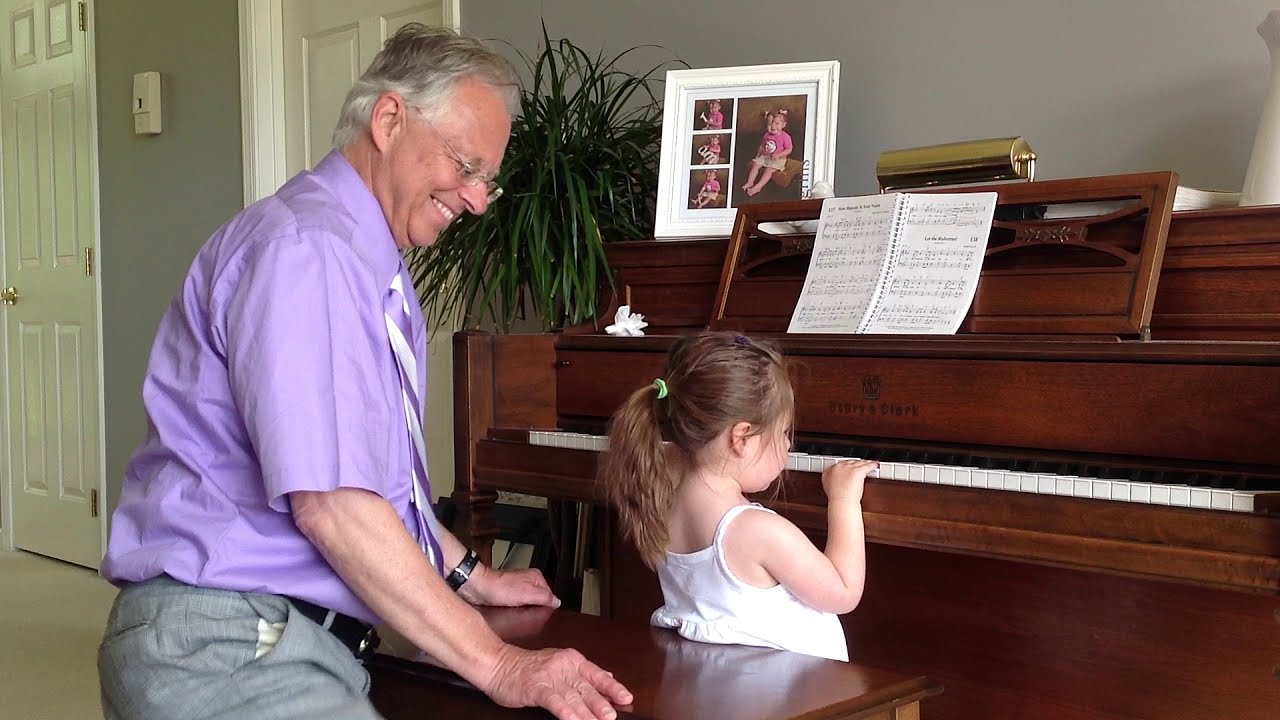In a cozy, gray-walled room, an older man with metallic glasses and gray hair stands beside a young girl who is playing on a classic dark brown upright piano. The man, dressed in a short-sleeved purple dress shirt with a white and purple striped tie and gray pants secured with a black belt, gently leans on the back of the dark brown wooden piano bench. He wears a warm, approving smile as he looks down at the girl, possibly his granddaughter.

The young girl, her hair pulled back into a ponytail with a green braid, is focused on the white piano keys. She stands before the piano in a white sleeveless shirt, her face just reaching the keys, and both hands poised on the instrument. Above the keys, an open book of piano music rests, and to its left sits a framed portrait on top of the piano. A vibrant green spider plant adds a touch of nature to the scene, positioned between the man's head and the portrait.

The photo, a horizontal 16 by 9 landscape image, captures the tender moment against the backdrop of two white doors in the far left corner of the room. A visible thermostat between the doors anchors the homey setting, making it a heartfelt depiction of a shared musical moment between generations.